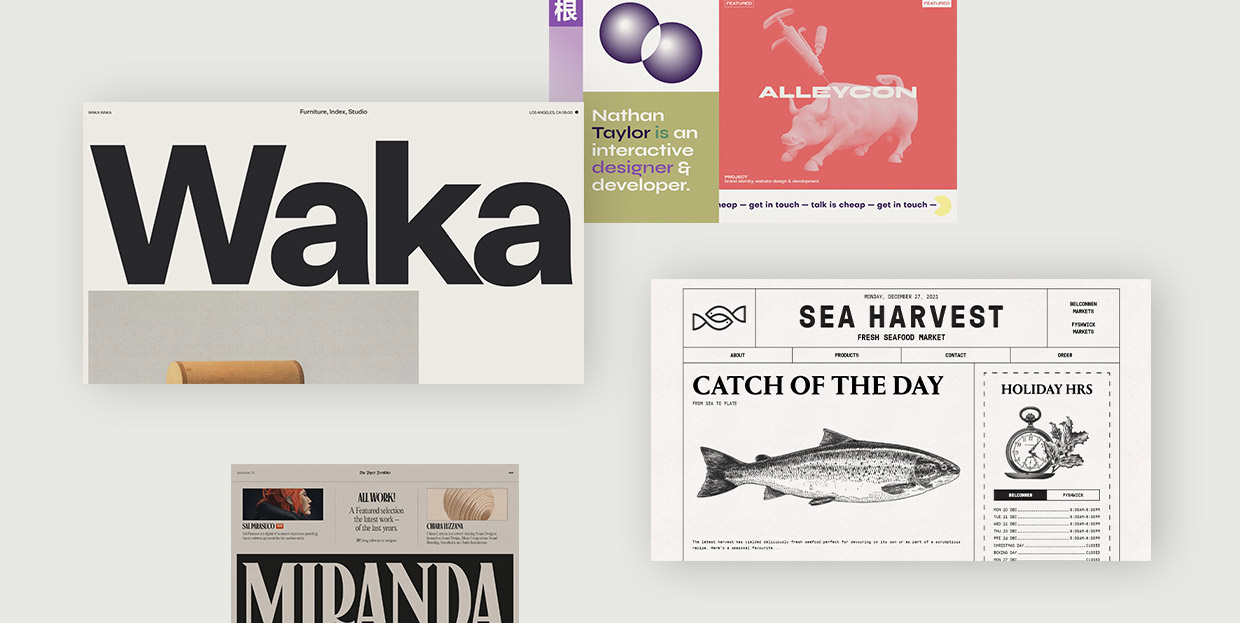The image is a collage of four distinct rectangular elements set against a gray background. 

1. **Top Left:** A white rectangle prominently displaying the word "W-A-K-A" in large black letters, with smaller unreadable text above and a partial brown photograph below.
2. **Top Right:** A detailed design labeled "Nathan Taylor is an interactive designer and developer," featuring two interlocking purple circles and a non-English character. To the right, a red square illustrates a pig being touched by a tool and captioned "Alicon."
3. **Bottom Right:** A black-and-white graphic for "Sea Harvest - Fresh Seafood Market," showcasing a fish with the phrases "Catch of the Day" and "Holiday Hours" next to a listing of operational times.
4. **Bottom Left:** A cut-out section of a magazine or newspaper cover with small pictures and text, highlighted by the word "Miranda" in white text against a black background.